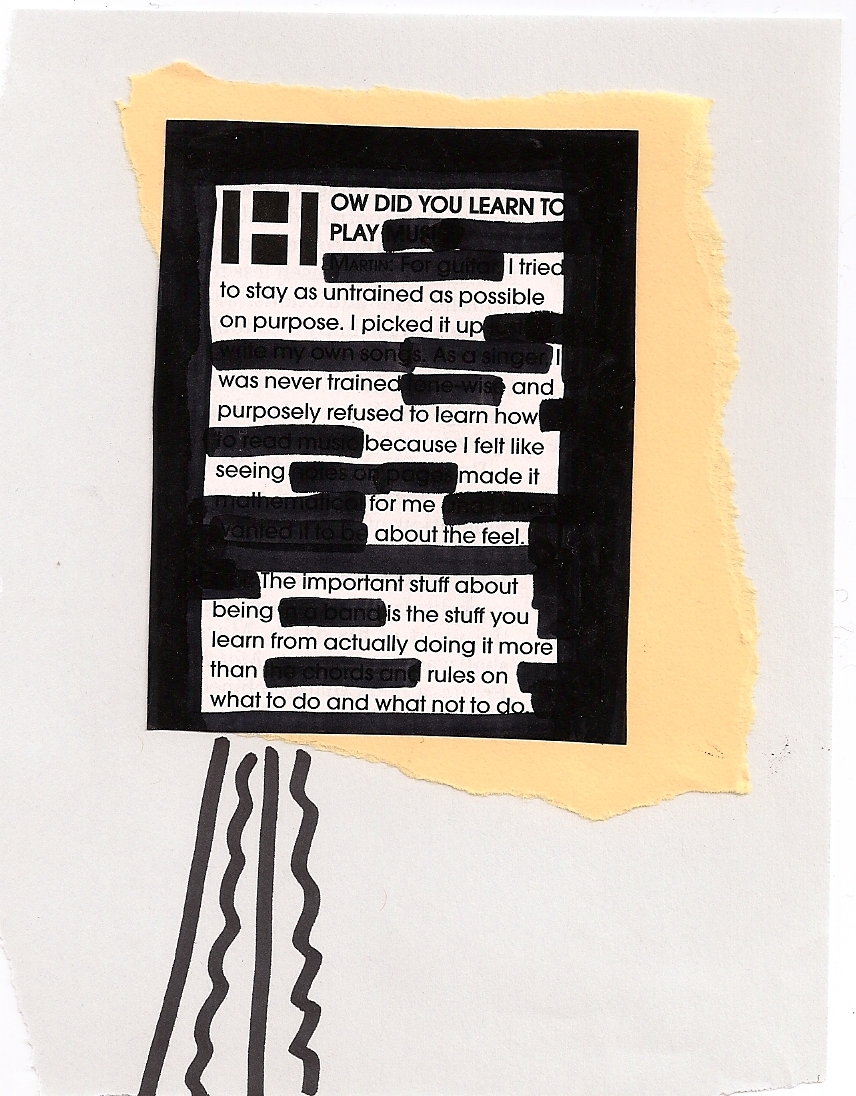The image depicts an artistic collage with a central black rectangle containing a piece of text that has been partially blacked out, creating a blackout poem. The text within the rectangle reads: "How did you learn to play? I tried to stay as untrained as possible on purpose. I picked it up, was never trained, and purposely refused to learn how, because I felt like seeing made it for me about the feel. The important stuff about being is the stuff you learn from actually doing it more than rules on what to do and what not to do." This rectangle is set against an abstract, orange-yellow paint smear on a white background, giving the impression of an art piece taped to a wall. Additionally, four black marker lines, both squiggly and straight, extend from the bottom of the rectangle. The combination of these elements creates a visually striking and thought-provoking composition reminiscent of modern art typically found in a museum.